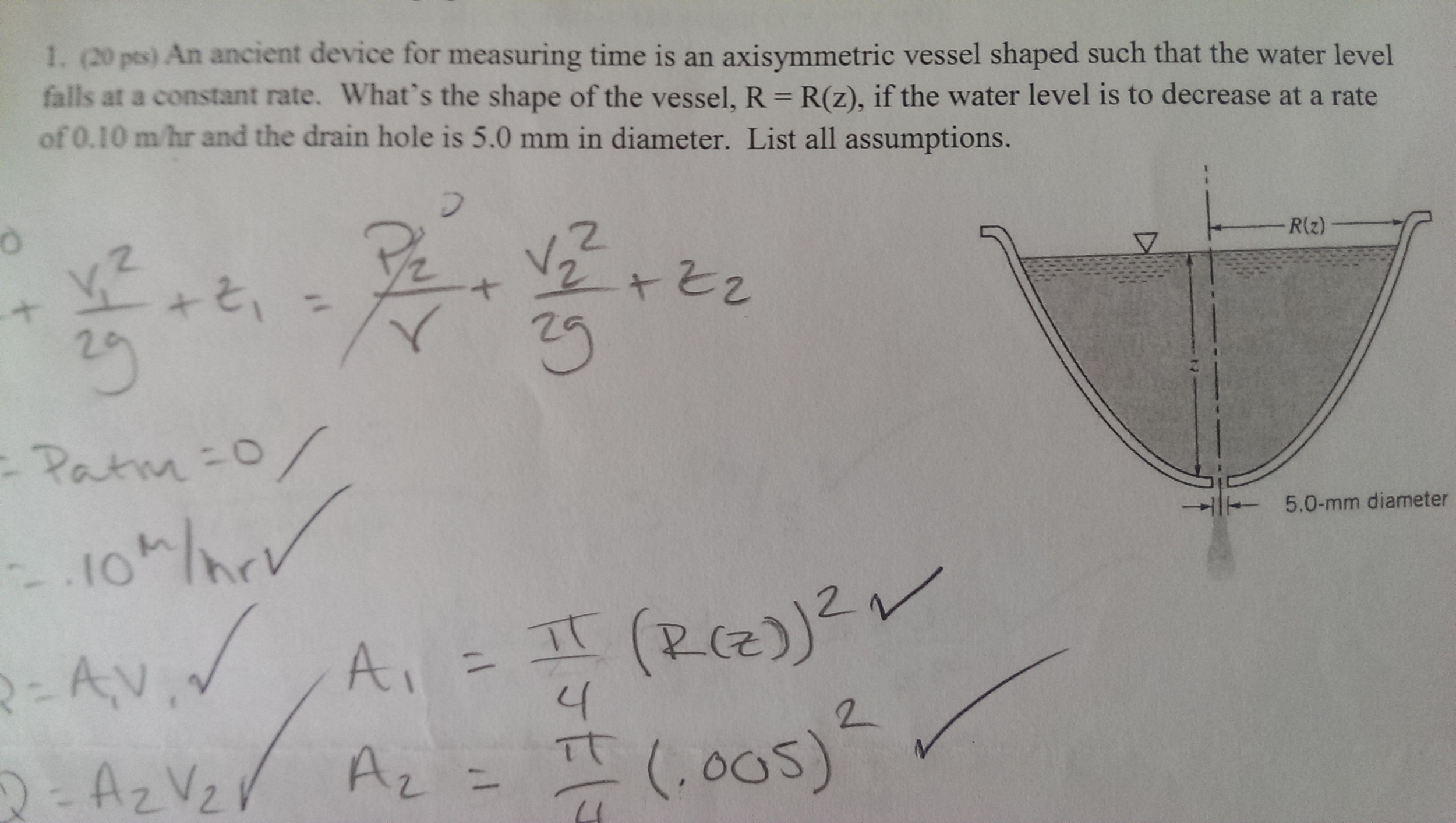This is a close-up photograph capturing a detailed math problem and part of a student’s handwritten solution. The problem, worth 20 points, appears to be from a test or assignment and reads: "An ancient device for measuring time is an axisymmetric vessel shaped such that the water level falls at a constant rate. What's the shape of the vessel? \( R = R(z) \). If the water level is to decrease at a rate of 0.10 meters per hour and the drain hole is 5 millimeters in diameter, list all assumptions." To the right of the text, there's a diagram illustrating the vessel with a small hole at the bottom, and annotations indicating the water level and key measurements. On the left side, the student's handwritten solution is shown, with all necessary equations and assumptions laid out in pencil. Several green check marks next to the steps indicate that the work has been reviewed and graded positively, suggesting that the solution is correct. It's not clearly specified, but the problem likely involves trigonometry or differential equations.